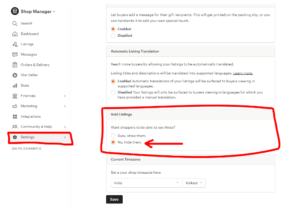The image displays a computer screen with a white background. On the screen, there are various panels and text options. The resolution is poor, making the text appear grayed out and difficult to read.

On the left side of the screen, there is a vertical panel topped with the words "Shop Manager" in dark letters. This panel contains approximately 12 to 13 selectable items. The very bottom item, which appears to be "Settings," is highlighted and enclosed within a red rectangle.

To the right of this vertical panel, a larger rectangle spans across most of the screen, approximately two to three times the width of the left panel. This section is divided into four horizontal panels, each with a gray bar at the top and a white area below containing selectable options.

In the top horizontal panel, there is some text and two selectable options. The top option is selected, indicated by an orange-filled circle, while the bottom option remains unselected with a white circle.

The second panel similarly contains text and two selectable options. The top option is again selected with an orange-filled circle.

In the third panel, there is a single line of text and two selectable options. The second option is chosen, marked by an orange-filled circle. A red arrow, starting from the right and pointing left, is drawn to indicate this selection. This panel is also outlined in red.

The fourth panel includes some text with a drop-down box for making selections, and a black response button with white letters in the middle, presumably saying "Save."

Overall, the screen displays a detailed interface for managing various settings and options, with specific selections and annotations highlighted in orange and red for clarity.